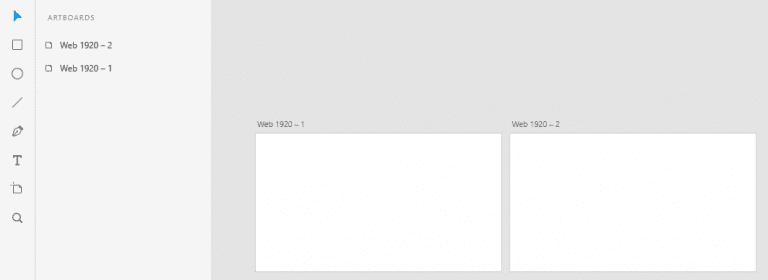The screenshot showcases an application interface with a sidebar on the left. The sidebar features a series of icons that appear to be tools, arranged vertically. Starting from the top, the first icon is a blue arrow, likely representing a share function. Below it, there is a square icon, followed by a circle, a diagonal line, the tip of a pen, a capital 'T', a cropping tool icon, and finally a magnifying glass indicating a search function. All icons, except the blue share arrow, are in a light gray color.

To the right of the icon toolbar, there's a vertical gray divider line. Adjacent to this line is the label "ARTBOARDS" in a small, light gray, all-caps font. Underneath the "ARTBOARDS" label, there are two checkbox options labeled "web 1920-2" and "web 1920-1," both of which are unchecked.

Further to the right is a larger, light gray rectangle, which seems to contain visual representations of different artboards. Inside this rectangle are two smaller white rectangles. The rectangle on the left is labeled "web 1920-1" in the top-left corner, while the one on the right is labeled "web 1920-2" in the same position.